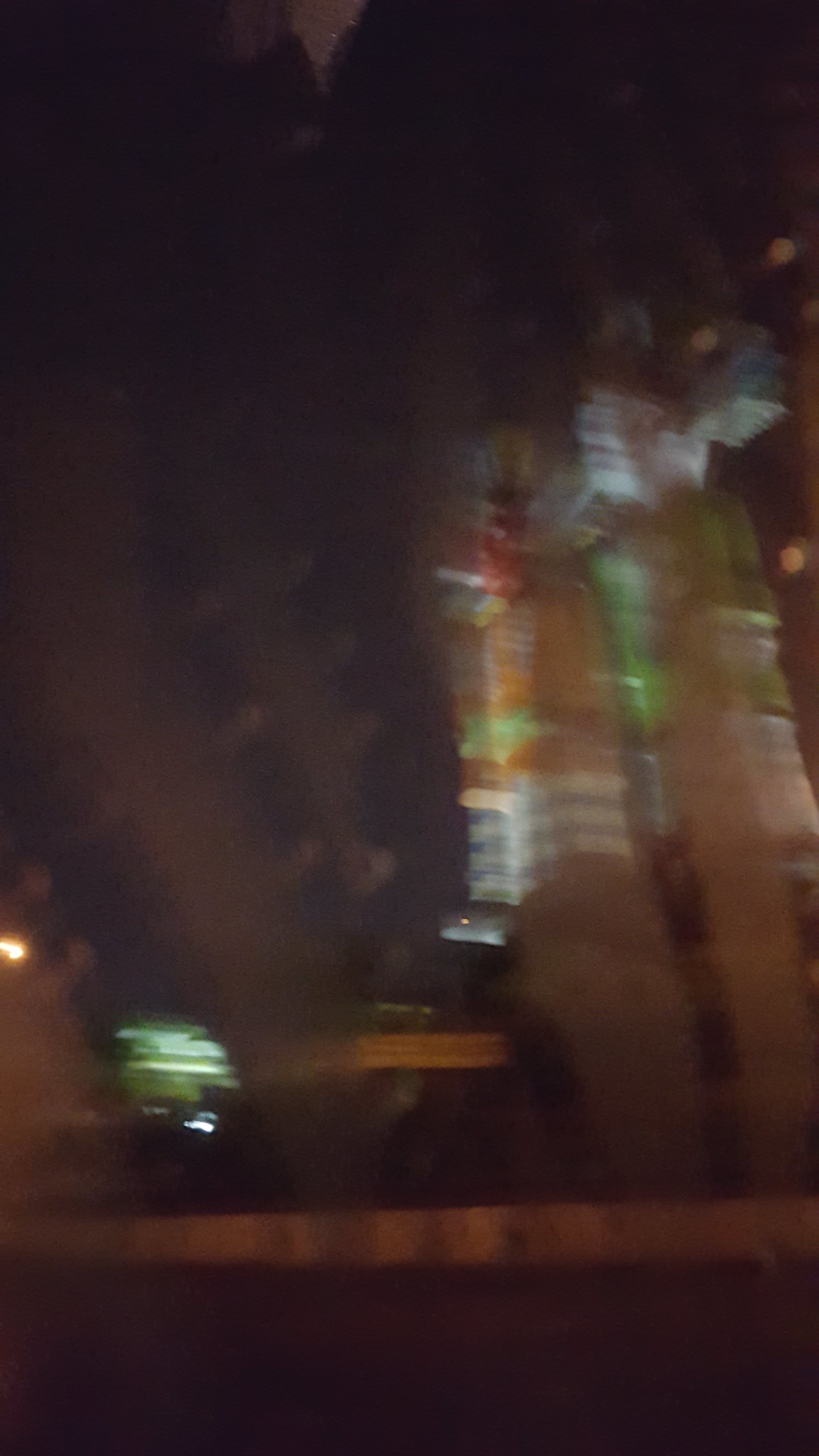A night-time cityscape captured in a slightly blurry photograph, showcasing an interstate road with a solitary vehicle, possibly a dark-colored truck, driving along the empty stretch. In the background, two illuminated high-rise buildings tower over the scene, their nature indiscernible but possibly office buildings or hotels. A distinct yellowish street light casts a soft glow on the surroundings, suggesting the photo was taken well after 9 p.m.